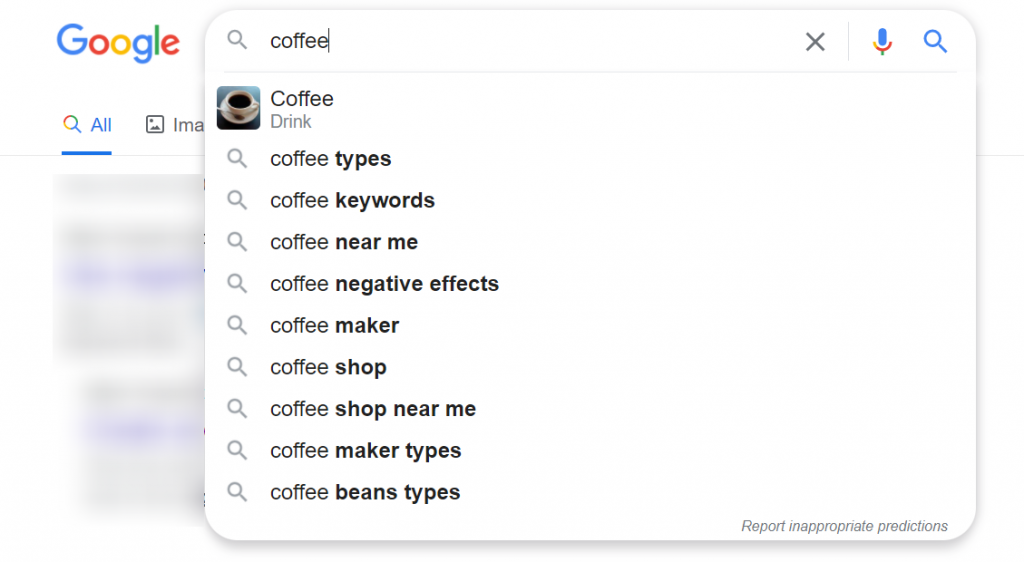**Detailed Caption:**

The image shows a Google search page featuring a partially completed search query for "coffee" in the search bar. The Google logo, displaying its usual blue, red, yellow, and green letters, is situated in the upper left corner. Below the search bar, a dropdown menu reveals several autocomplete suggestions related to the term "coffee." These suggestions include "coffee," "coffee types," "coffee keywords," "coffee near me," "coffee negative effects," "coffee maker," "coffee shop," "coffee shop near me," "coffee maker types," and "coffee beans types." Each suggestion is accompanied by a small magnifying glass icon indicating a search option.

To the right of the search bar are the microphone icon for voice search, an 'X' symbol to clear the search, and the search button itself. Below the search bar, slightly blurred text can be seen, possibly representing search results. The upper left section beneath the Google logo features partially visible buttons labeled "All" and "Images" for filtering search results. The page has a clean, white background, ensuring the search elements stand out clearly. Additionally, a "Report inappropriate predictions" link is located at the bottom right-hand corner of the page.